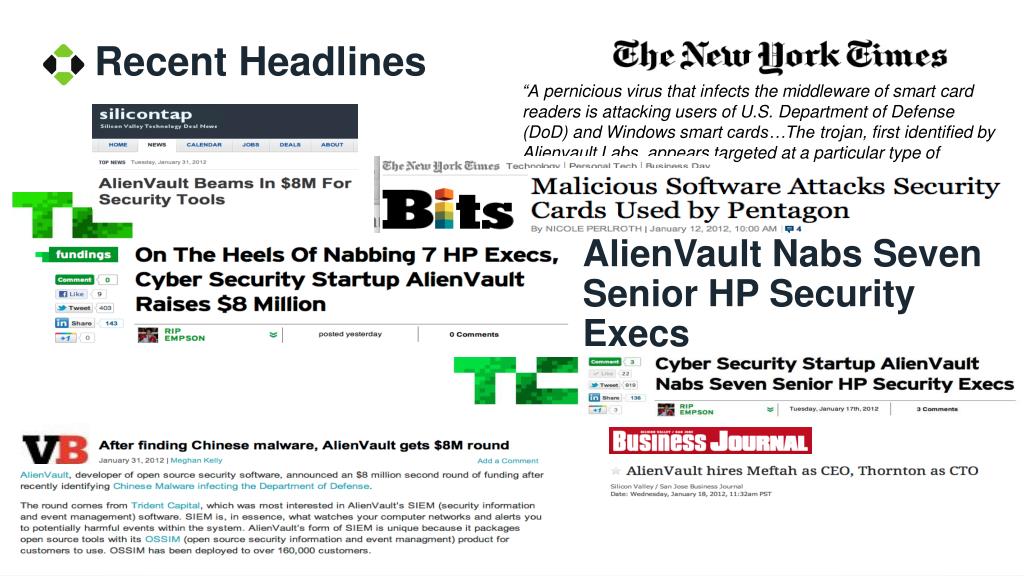**Descriptive Caption:**

The image features a white background adorned with various headlines printed in black. In the upper right-hand corner, a black and green diamond-shaped logo accompanies the text "Recent Headlines". 

Directly beneath, one headline prominently states: "Silicone Tap Alien Vault Beams in 8 Million from Security Tools".

On the right side, a headline from The New York Times reads: "A pernicious virus that infects the middleware of smart card readers is attacking users at the U.S. Department of Defense and Windows smart cards. The Trojan first identified in Alien Vault lambs appears targeted at a particular type of..." (the text cuts off).

Below that, another New York Times headline states: "Bits: Malicious software attacks security cards used by Pentagon".

Further down, a headline from Alien Vault reports: "Alien Vault Namps Seven Senior HP Security Execs".

Adjacent to this, a green TC logo captions: "Cybersecurity startup Alien Vault namps seven senior HP security execs".

On the left side of the image, a bold headline reads: "On the heels of namps seven HP execs, cybersecurity startup Alien Vault raises 8 million".

Finally, the VB logo (with "V" in black and "B" in red) displays: "After finding Chinese malware, Alien Vault gets 8 million dollar round. Alien Vault, developer of the open-source security software, announced the 8 million second round of funding after recently identifying Chinese malware infecting the Department of Defense". Additionally, it notes: "Alien Vault hires Mefta as CSO or CEO and Thornton as CTO".